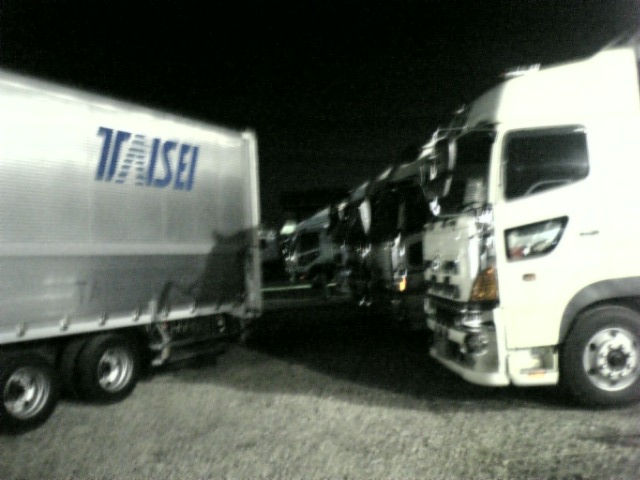This is a nighttime color photo depicting a lineup of semi-trucks in an outdoor parking lot with a gray asphalt ground. To the left of the image, there is a silver metallic truck, distinguished by its blue logo that appears to read "TAISEI." The "A" in the logo is composed of horizontal lines, and the "T" features an additional line cutting through it. The black tires of this truck are clearly visible. On the right side of the image, there are several white trucks, each visible from the front, showcasing the driver cabins and black tires. These trucks form a neat row, casting shadows to the right, which accentuates the dimly lit, slightly grainy and blurry quality of the photograph. The image captures the industrial ambiance of the lot, with the silhouettes of the trucks standing starkly against the nearly black night sky.